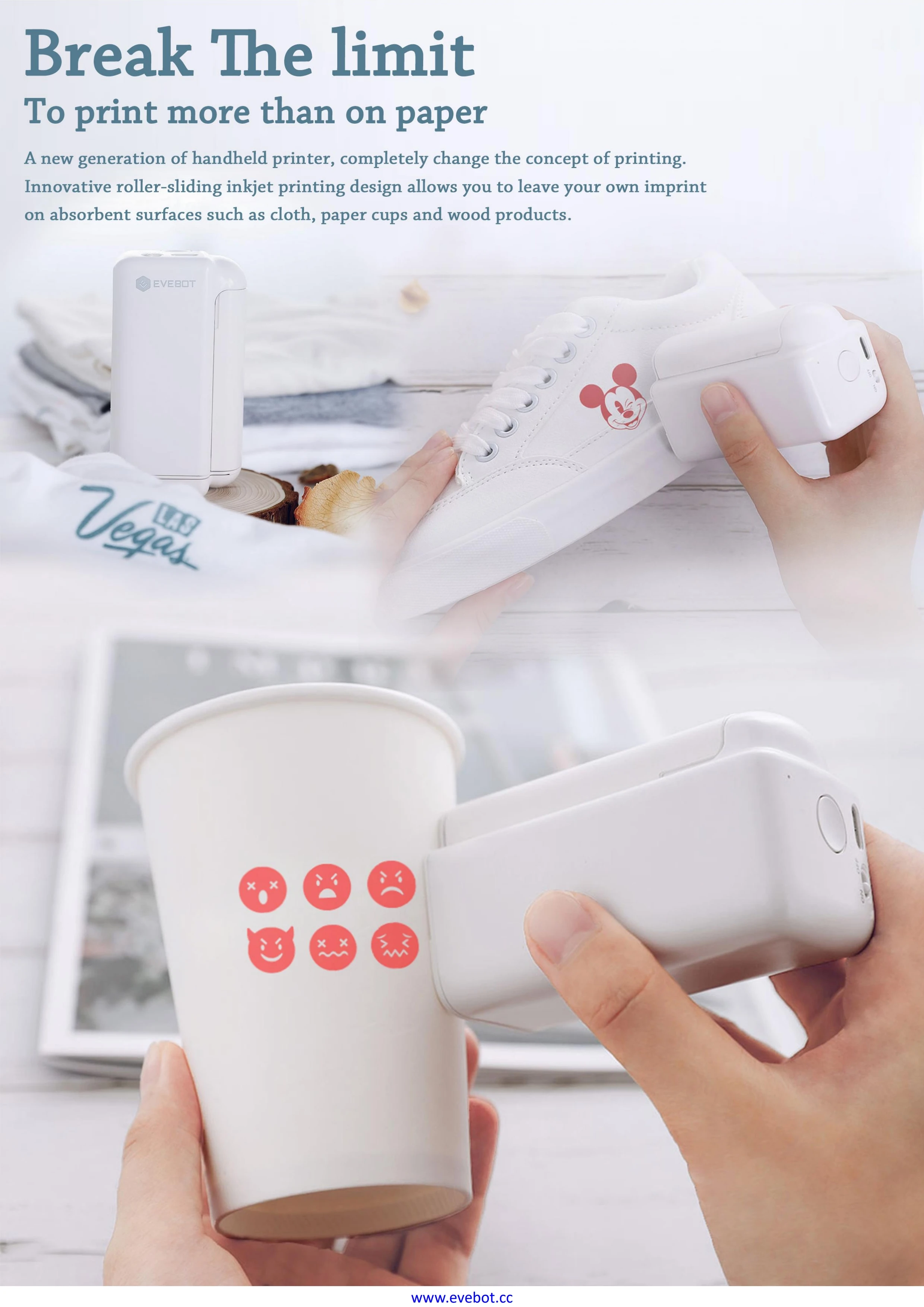This advertisement showcases a cutting-edge handheld printer on a varying light background from white to gray. At the top, in greenish-blue ink, it states, "Break the limit to print more than on paper. A new generation of handheld printer completely changed the concept of printing." Highlighting its innovative roller-sliding inkjet design, the ad emphasizes its capability to print on absorbent surfaces like cloth, paper cups, and wood products.

The ad features several images demonstrating its versatility: one shows the device upright with stacks of cloth behind it, illustrating its use on textiles. Another shows an individual holding a white sneaker and using the printer to imprint a light reddish image of Mickey Mouse on it. Additionally, the device is depicted on a stand beside a printed "Las Vegas" graphic. In a third example, a woman holds a white paper cup in front of framed art, showcasing printed faces ranging from smiley to devil-like emojis on the cup. The small, white rectangular printer is described as having a protrusion on top, effectively used to create various imprints on diverse materials, suggesting the brand "EveBot" and directing viewers to www.evebot.cc for more information.